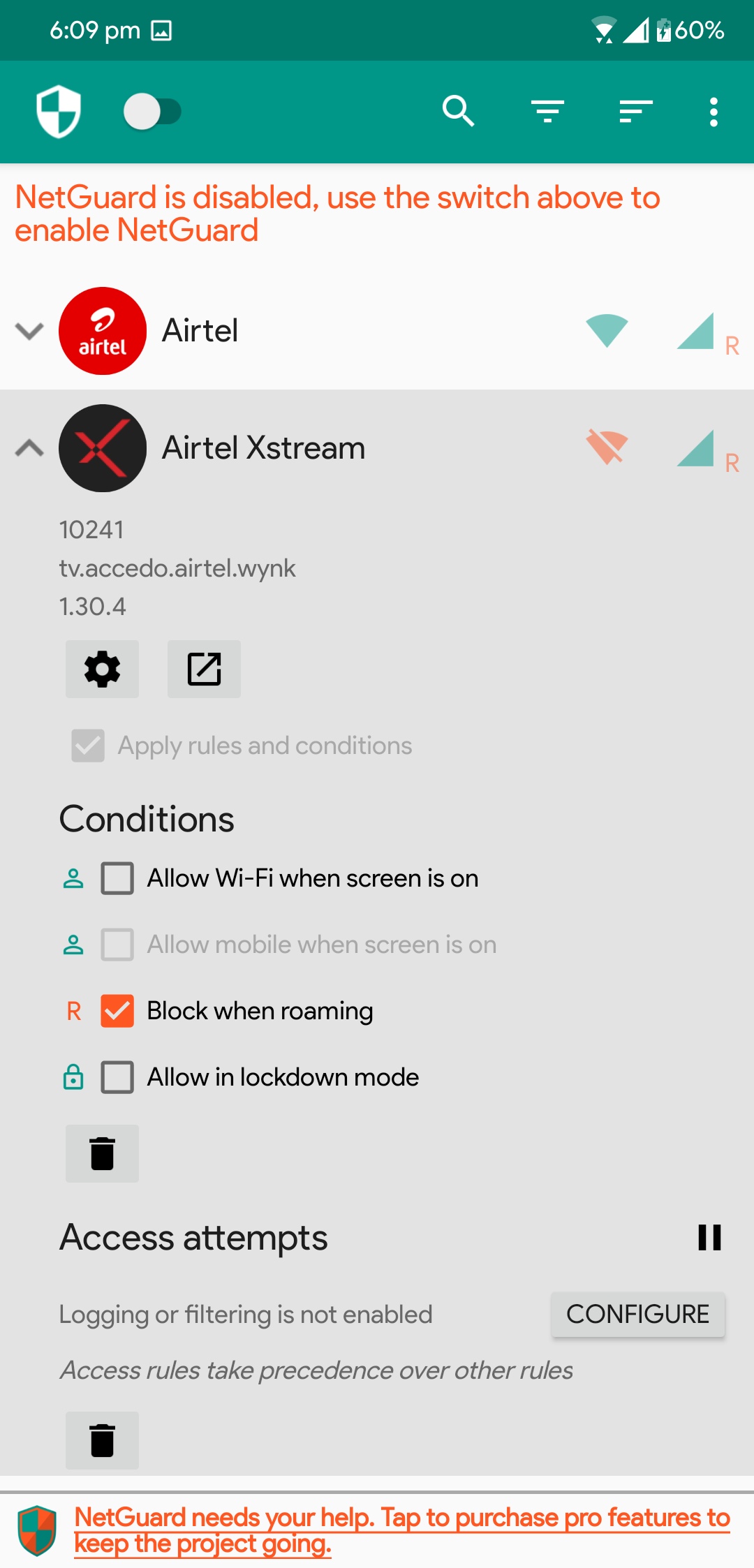This screenshot depicts the settings page of an application or service interface. At the top of the page, a green bar spans across the screen. On the left side of this bar, there is a shield icon paired with a white toggle switch. On the right side, the bar features several icons in the following order: a search icon, a filter icon, an icon resembling a statistics bar, and an information icon.

Beneath the green bar, there is a prominent message in orange text on a white background. The text states, "NetGuard is disabled. Use the switch above to enable NetGuard." Directly below this message resides a drop-down menu displaying "Airtel" within a red circle, accompanied by the text "Airtel" positioned to its right. Further to the right, there are two icons: a Wi-Fi icon and a signal strength icon.

Following this section, there is a gray area containing additional details. Within this gray section, there is an upward-pointing arrow and a black circle with a red 'X’ inside it, labeled as "Airtel Extreme." Additionally, there is an orange Wi-Fi icon with a cross over it and a green signal strength icon.